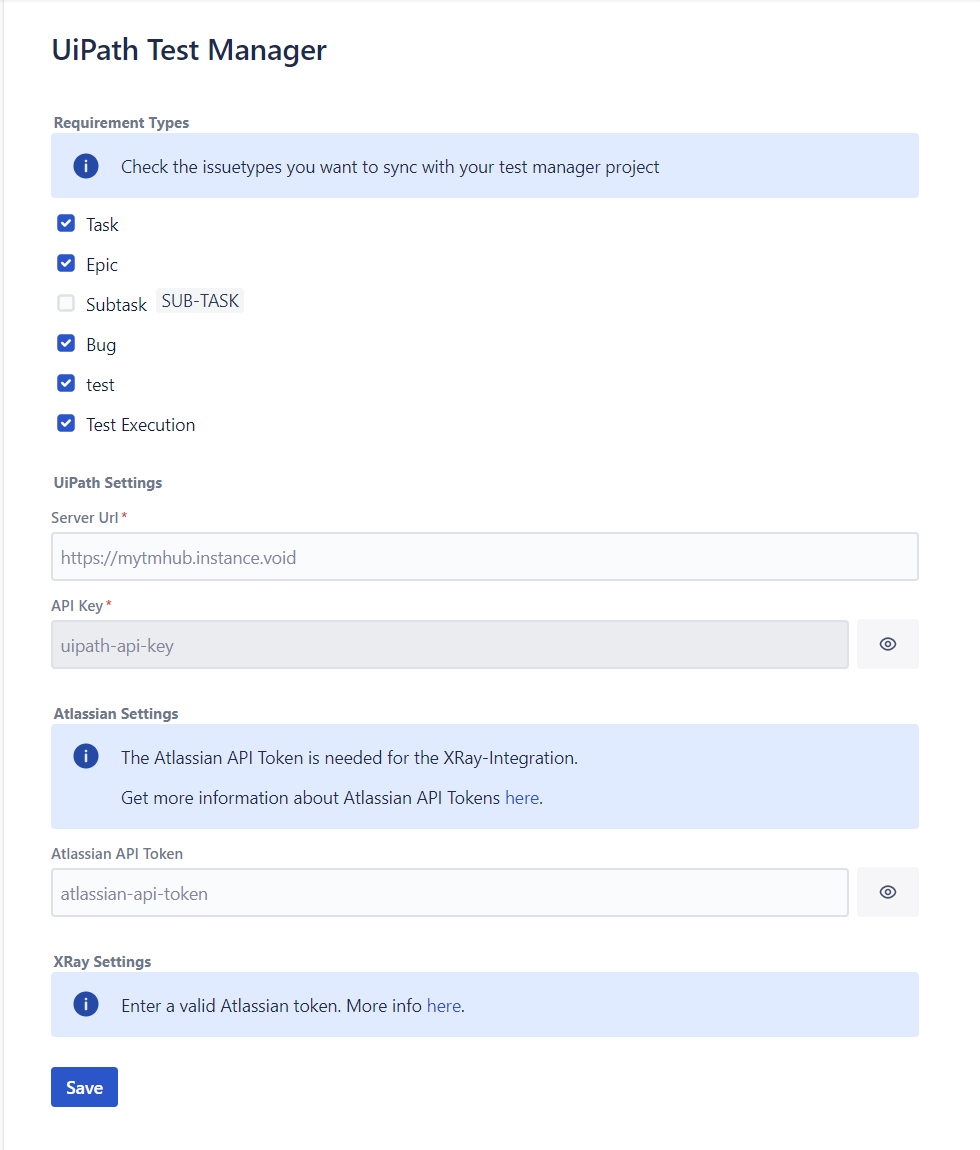This screenshot is taken from a website interface titled "UiPath Test Manager." At the top, it prominently displays the title followed by various configuration options. Below the title, there's a section labeled "Requirement Types" with an exclamation mark, instructing users to select the issue types they want to sync with their test management project. The selectable options include Task, Epic, Subtask, Bug, Test, and Test Execution, with all options selected except for "Subtask."

Further down, the interface is divided into different settings sections. The first section, "UiPath Settings," displays a field for the server URL, which is set to "https://mytmhub.instance.void," and another field for the API key, displayed as "UiPath-API-Key."

Following this, the "Atlassian Settings" section indicates that an Atlassian API token is needed for X-Ray integration, with a link provided for more information about acquiring Atlassian API tokens. This section includes a field labeled "Atlassian API Token," shown as "Atlassian-API-Token."

The final section, "X-Ray Settings," prompts the user to enter a valid Atlassian token, with a link for additional information. The screenshot concludes with an option to save the configured settings.

Overall, the screenshot provides a detailed view of the settings and configuration options for synchronizing various project management tasks and integrating with Atlassian tools within the UiPath Test Manager interface.